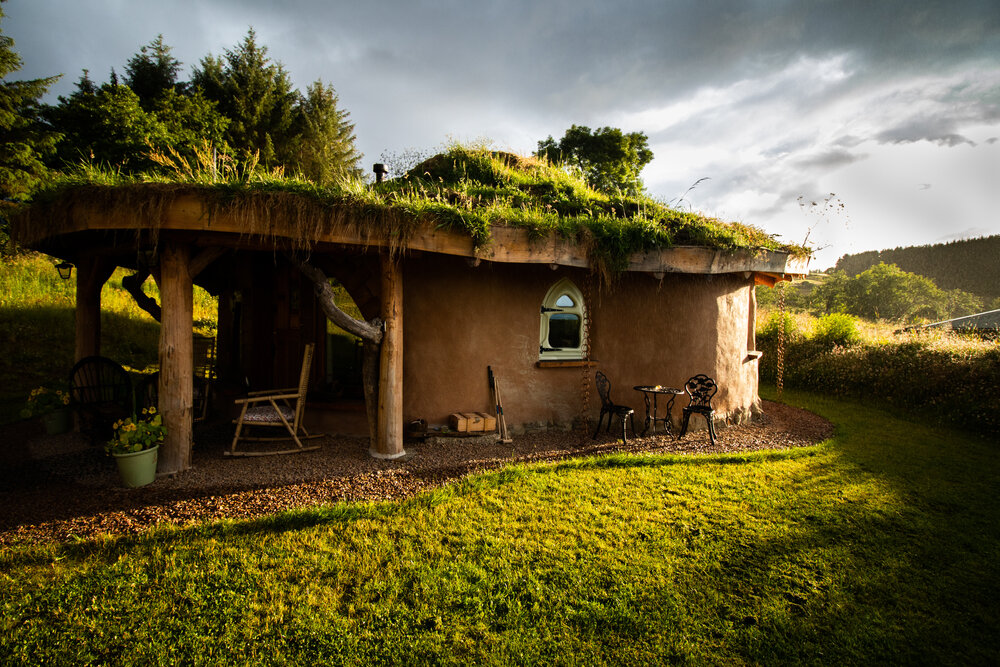This image features a unique, small, one-story dwelling set in a vibrant, green landscape. The structure has a rustic, earthy texture, possibly made of adobe or smoothed-over mud, giving it a homemade appearance. Its distinctive flat roof is adorned with lush, green grass and vegetation, some of which drapes over the edges, creating the impression of a living roof.

The front of the house is characterized by an overhanging porch, supported by a trio of rounded, wooden pillars at each corner. Beneath this extended roof, a rocking chair is positioned to the left, and a small black iron table with two matching chairs is set to the right. Additionally, a couple of potted sunflowers and other flowers in containers add splashes of color to the otherwise earthy tones.

The backdrop consists of trees and rolling hills under a dramatically overcast sky. The cloud cover is heavy and dark at the top, transitioning to a lighter gray towards the horizon, suggesting impending rain or a storm clearing up.

The overall atmosphere is one of rustic tranquility, with the eclectic greenery on the roof harmonizing with the surrounding natural environment. It's a serene scene that feels both homemade and harmoniously integrated with nature, framed by the lush greenery and the moody sky above.